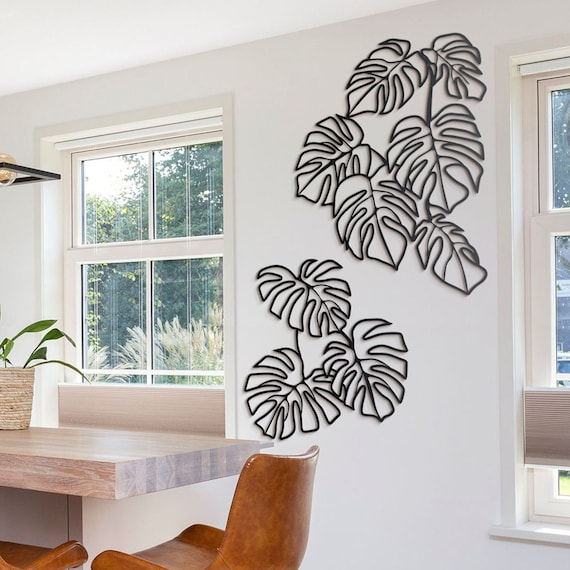The image showcases the interior of a house with white walls, highlighting a corner that could be part of a kitchen or a cozy nook. The focal point of the decor is a set of stenciled or outlined metal or plastic leaves arranged on the wall. There are nine leaves in total, appearing as hollow or stripped silhouettes, and they are black in color. These decorative leaves are positioned above a wooden table—potentially used as a dinner or bar table—with a cherry wood finish. The table holds a potted plant in a bucket that might be crocheted or made of clay, with green, floppy leaves. Surrounding the table are wooden chairs, one prominently visible and another partially in view. The corner is well-lit by a rustic metal light fixture featuring an old-style incandescent bulb. Nearby, two windows with slightly raised blinds allow a clear view of tall grass and trees outside, adding to the serene ambiance of the space.